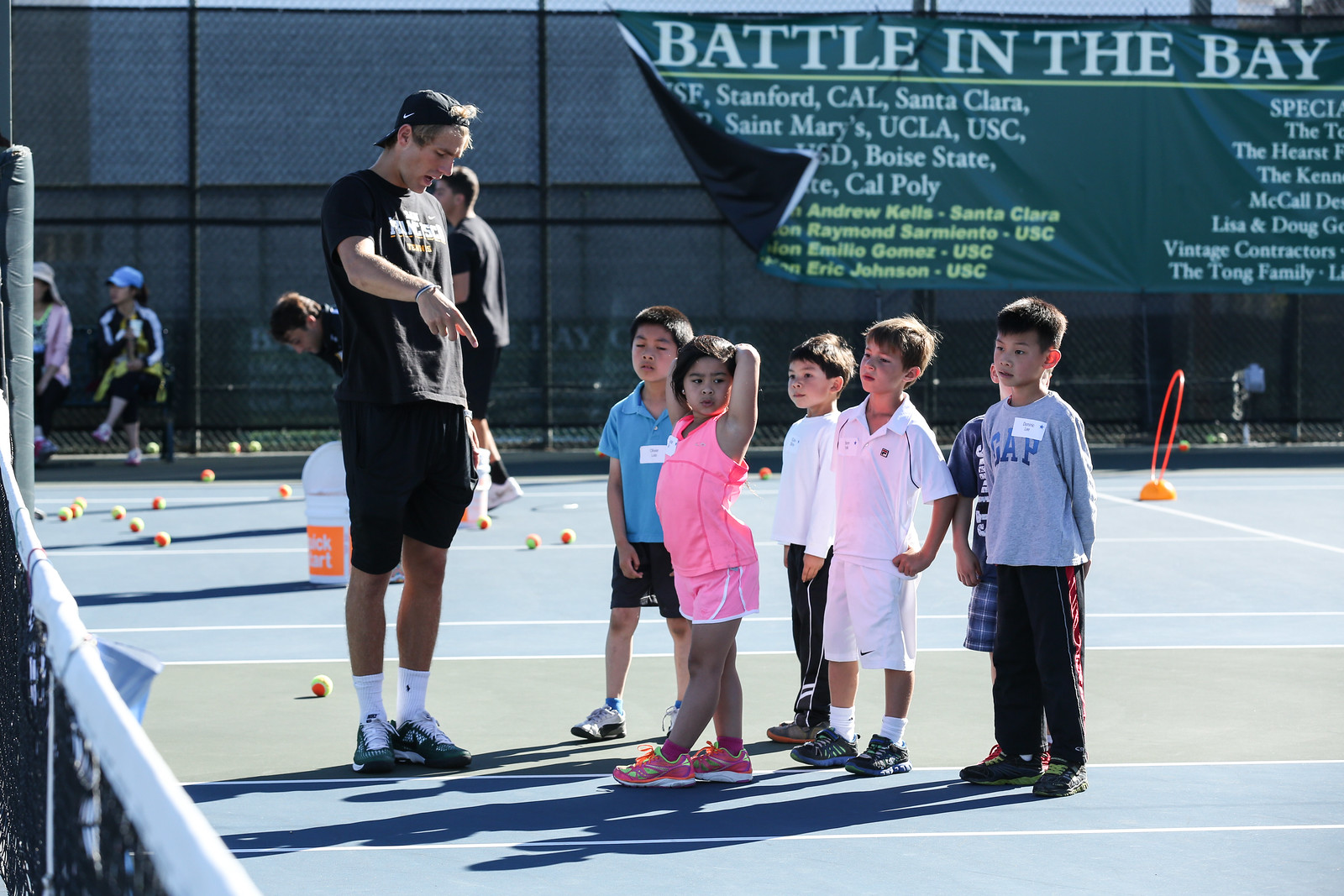This detailed photograph captures a lively tennis lesson taking place on a multi-court tennis complex. The court is predominantly blue and green, scattered with multiple tennis balls hinting at an ongoing practice session. Central to the image is a group of young children, approximately six or seven years old, gathered attentively around a coach. The group consists of five boys with short-cropped hair and one girl dressed in a pink shirt and matching shorts, standing out with her longer hair. The children, wearing a mix of colorful outfits ranging from blue, white, to gray, are focused on the instructor.

The coach, a young man in his 20s, is donned in an all-black athletic outfit, accented only by his white socks and a black Nike cap worn backwards. He is animatedly pointing towards something, likely giving instructions to the eager young learners. 

In the background, a few adult women sit and observe the session, adding to the community feel of the scene. Behind them, a large banner attached to a tall chain-link fence reads "Battle in the Bay," promoting a tennis event that features colleges such as Stanford, Cal, Santa Clara, St. Mary's, and UCLA. The banner, green with yellow and white text, and the chain-link fence provide a clear yet slightly obscured backdrop that grants a sense of privacy to the area. Overall, the photograph blends the elements of a structured sports lesson with the casual atmosphere of a local tennis court.